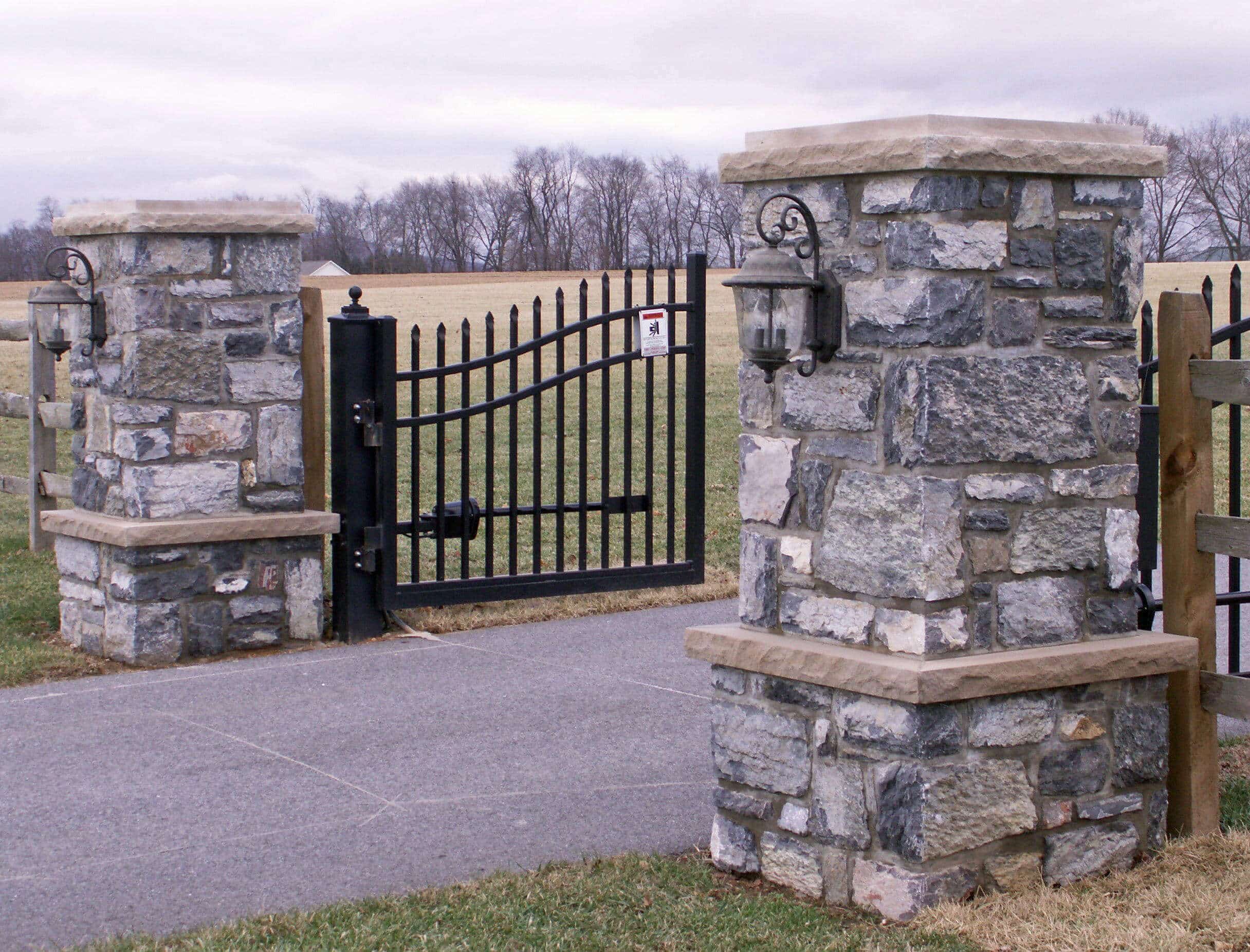The photograph depicts the entrance to a property, featuring a central driveway flanked by imposing stone pillars composed of gray, white, and dark gray bricks. Each pillar is crowned with a gray slab and adorned with wrought iron carriage lights. A black wrought iron gate, presently open but capable of closing, spans the driveway. To the right of the driveway, a brown wooden fence extends into the scene. The surrounding grass appears brown, suggesting a seasonal change, and a small white and orange security sign is visible on one of the automatic gate apparatuses. The background reveals a vast field with bare trees and a cloudy, dreary sky, hinting at winter or cold weather conditions.